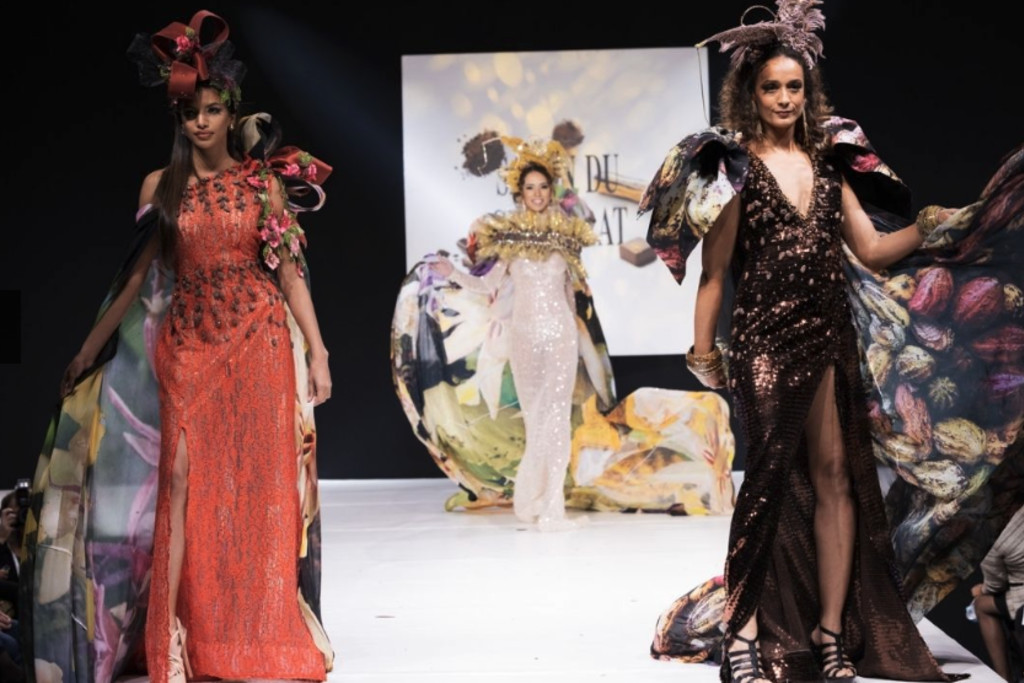This landscape fashion photograph captures a dynamic runway scene with three striking women on a brilliantly lit white stage set against a black background. The primary focus is on the two women closest to the camera, while a third woman is positioned further back near the edge of the stage, appearing smaller in comparison. 

On the left, the first model is a darker-skinned woman with long black hair cascading past her shoulders. She dons a slightly orange-tinged, sequined red dress adorned with brown textured cloth accents near the chest and waist, and a florally printed, multi-colored cape drapes around her, adding movement and flair. Her look is complemented by a large, ribbony red hat, and she gazes intensely over the viewer's left shoulder, her expression serious.

The model on the right, also close to the camera, sports a dramatic dark purplish or black v-neck dress that exposes her left leg up to the upper thigh. Her dress sparkles with light purple sequins, and she accessorizes with a flamboyant pink hat with floral puffs. Her shoulders are bare, and she wears high-heeled shoes with straps across the top. A multi-colored, wing-like cape extends behind her, adding a touch of theatricality. She looks off to the right, past the audience.

In the center, far back on the stage, stands a model in a form-fitting, silvery white sequined gown that flows to her feet. Dark-haired and smiling directly at the camera, she exudes confidence and elegance. Her attire includes a golden, puffy accessory around her shoulders and a matching golden headdress. A vibrant, multi-colored floral cape billows behind her, enhancing the ethereal quality of her outfit.

Together, these three women present a visually stunning tableau of contrasting yet harmonious fashion statements, each adorned with intricate details and vibrant colors, illustrating the creativity and drama of high fashion on display.